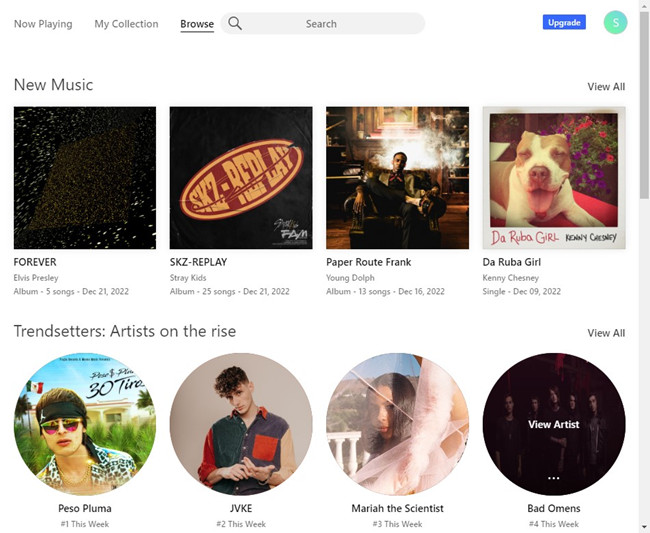This image showcases the interface of a music streaming service webpage. The top navigation bar includes key sections, labeled from left to right as: "Now Playing," "My Collections," and "Browse"—with "Browse" being bolded and underlined. Additionally, a search icon is located toward the center, while on the far right, a blue "Upgrade" button and an aquamarine circle with an "S" initial are visible.

The webpage prominently features a section titled "New Music" on the far left side, displaying four notable album covers:

1. **Forever** by Elvis Presley - Released on December 21, 2022.
2. **SKZ Replay** by Stray Kids - Comprising 25 songs, released on December 21, 2022.
3. **Paper Route Frank** by Young Dolph - Featuring 13 tracks, released on December 16, 2022.
4. **Da Rubagirl** by Kenny Chesney - Released on December 9, 2022.

Adjacent to these album covers is a vivid Polaroid image of a pitbull lounging on a red cushion, framed by purple and red flowers in the background.

The second section, titled "Trendsetters, Artists on the Rise," highlights emerging artists with circular portrait images. The artists featured are:

1. **Peso Pluma** - A man wearing a black Air Jordan bandana and shades.
2. **JVKE** - A young artist with a trendy 'broccoli' haircut, dressed in a uniquely split collared shirt that is half green and half violet, adorned with an orange front pocket on the violet side.
3. **Maria The Scientist** - Another youthful musician, sporting straight, shoulder-length hair parted in the middle and a pink lace scarf.
4. **Bad Omens** - A rock band, represented by its collective image.

This detailed and vivid layout illustrates the wide array of music and artists available on the streaming service, providing both visual and textual emphasis on the latest releases and emerging talents.